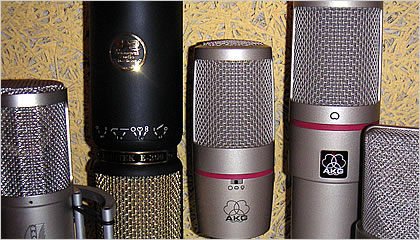This photograph showcases five condenser microphones meticulously aligned from left to right on a yellow and gray straw-textured surface. Each microphone features a distinct design, with four of them displaying a sleek, silver or gray metallic finish and one boasting a striking black handle with a gold mesh head. The silver and gray microphones have a metallic mesh pattern where sound is captured, creating a detailed and vintage appearance, akin to those used by singers. Among the silver microphones, two are branded with red lines and the name "AKG" prominently displayed on their solid metal bases. The most visually distinctive is the black and gold microphone, featuring a black handle and a gold mesh head, accented with a shining gold circular logo in the middle.